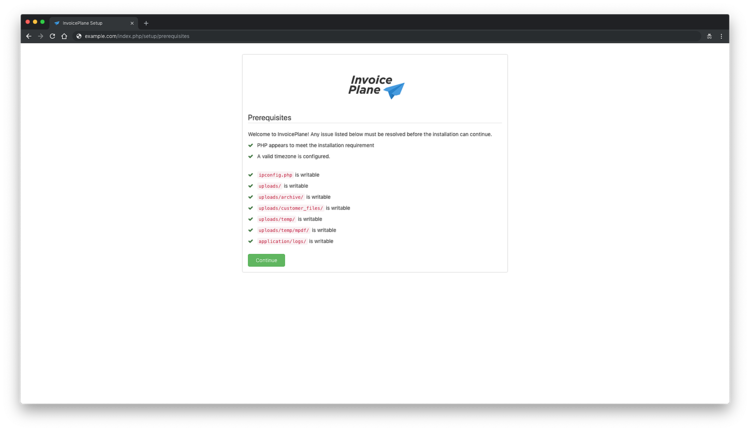The image is a horizontally rectangular screenshot of a computer screen. At the top of the screen, there is a narrow black banner populated with various, though mostly indistinguishable, emojis. At the far left of this banner, discernible navigation buttons such as back, forward, and refresh can be seen, albeit very small. Below the banner, there is a single browser tab, next to which an address bar containing an unreadable web address is positioned. To the far right of the address bar, there appears to be an icon indicating incognito browsing, but its small size makes it hard to confirm.

The majority of the screenshot features a white background with a centered, light gray-outlined box. Prominently in the middle of this box is the "Invoice Plane" logo, accompanied by a blue paper plane icon. Below the logo, the word "prerequisites" is visible, followed by a vertical list. Each item in this list is marked with green check marks, though the specific text of the items on the list remains unreadable.